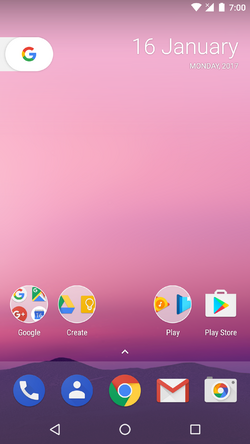This image features a screenshot of a cell phone home screen. At the top of the screen, the status bar displays signal strength, battery level, and the current time. Beneath the status bar, the home screen has a pink background. In the upper right corner, the date is prominently displayed in white text, reading "16 January, Monday 2017." On the left side, there is an icon for Google, suggesting that the Google suite can be accessed by swiping. Near the bottom of the screen, several app icons are visible. Starting from the left, the icons include Google, Create, Play, and Play Store. Below these icons, a row of essential app icons is displayed: phone calls, contacts, Chrome, Gmail, and photos on the far right.